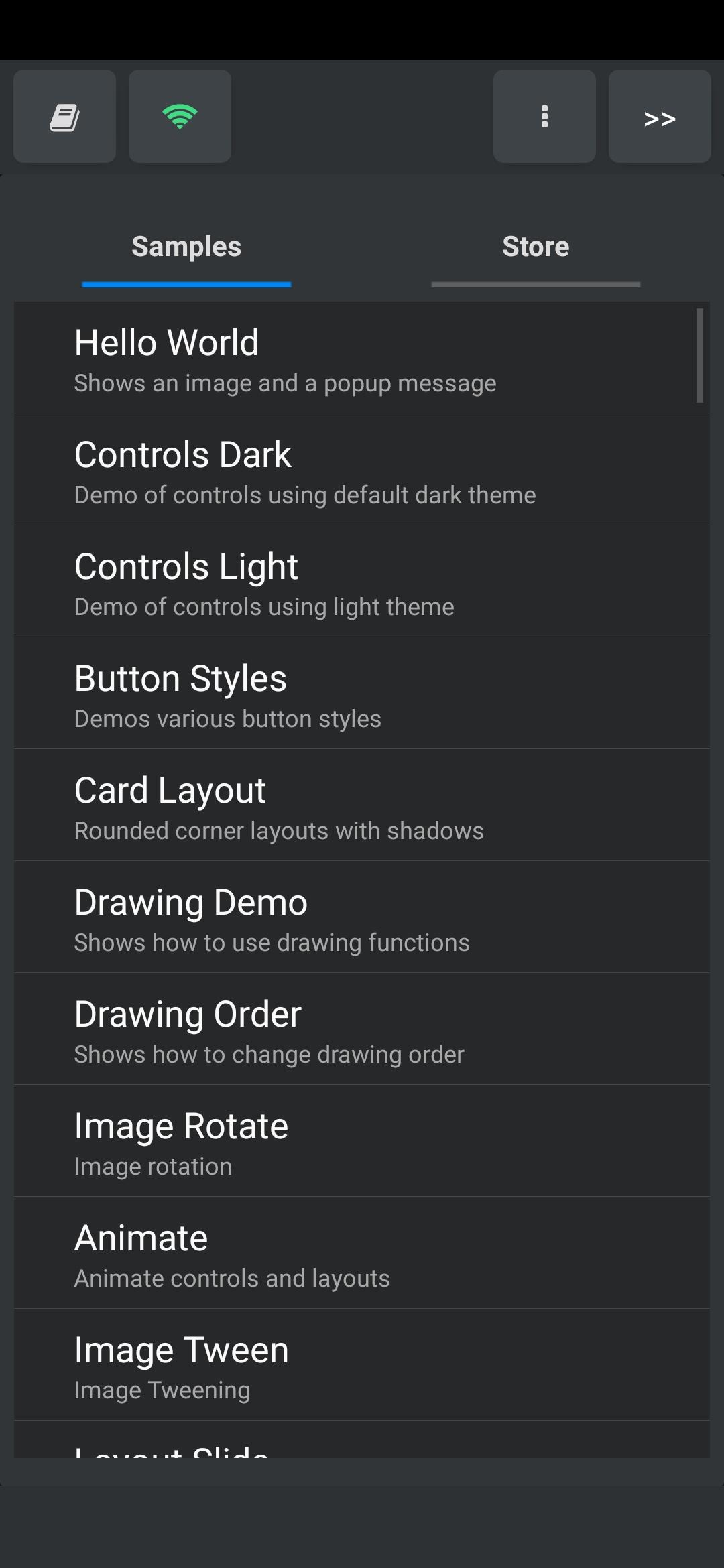This image is a screenshot from a coding or image control application, which may resemble platforms like Scratch. The screenshot prominently features a list of commands under the subtitle "Samples," which is underlined with a bright blue line for emphasis. 

The first command listed is "Hello World," and it is described as showing an image accompanied by a pop-up message. Following this, there are several other commands including "Controls Dark," "Controls Light," "Button Styles," "Card Layout," "Drawing Demo," "Drawing Order," "Image Rotate," "Animate," "Image Tween," and "Layout Slide." Each command has a brief description underneath, explaining its function.

The background of the screenshot is a combination of grey and black, providing a neutral backdrop that allows the commands and descriptions to stand out clearly. The design and structure of the interface appear user-friendly and are likely intended to assist users in navigating and utilizing various functions of the application effectively.